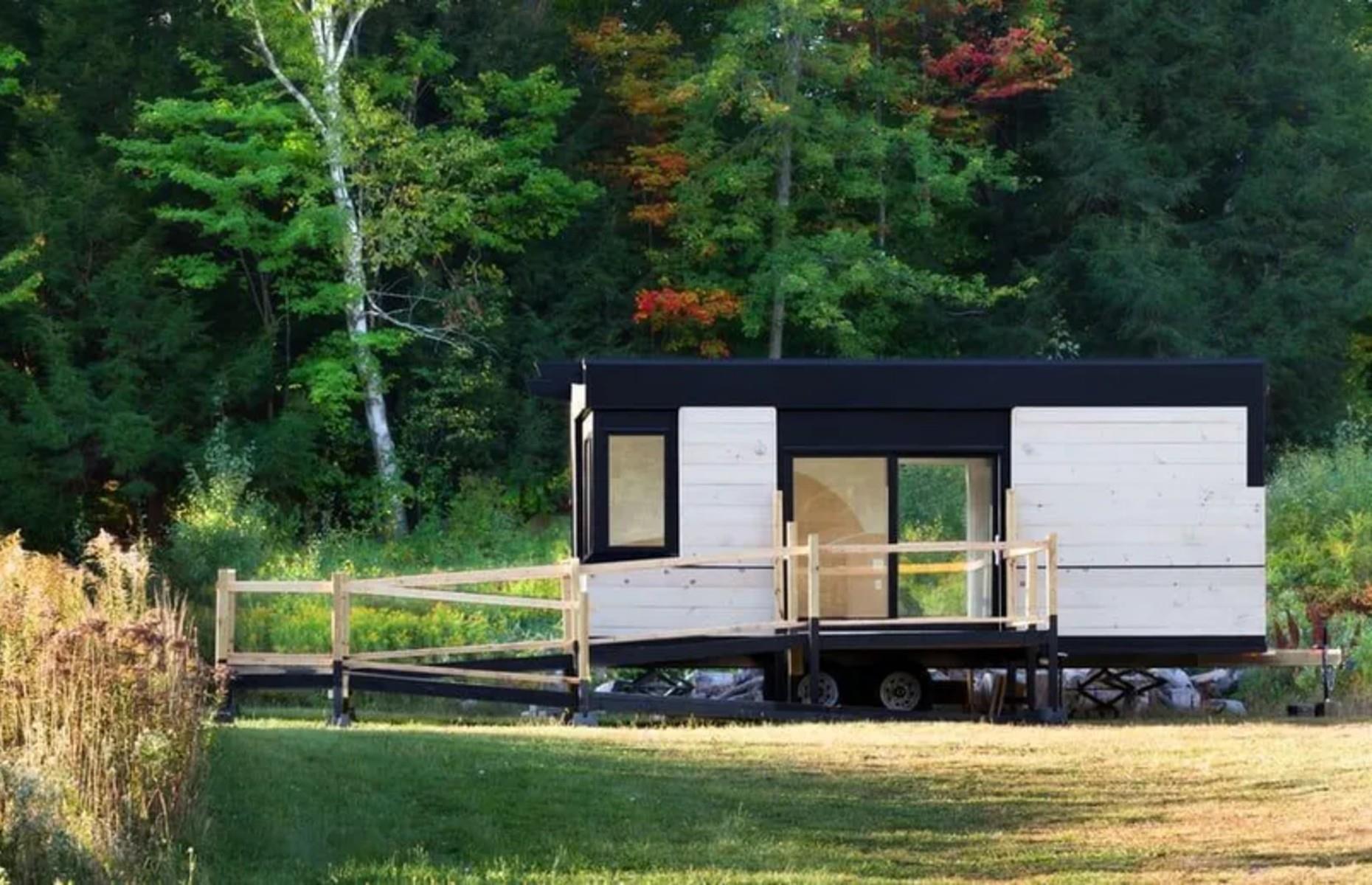This color photograph captures a small, white trailer with a dark blue or black roof, set in a grassy field transitioning into a forest. The trailer, situated on four wheels with additional support structures underneath, features unpainted wood siding and a large open space at the front. A sliding glass door is centered on one side, flanked by a narrow vertical window. A wooden ramp with a steel base and wooden railings leads up from the front entrance, turning before continuing up to the open entryway. The surrounding area includes a mix of green and brown grass, shadows, and various plants. The forest in the background displays a rich tapestry of greenery interspersed with red and orange leaves, indicating the onset of fall. Visible are some white tree trunks and a mix of pine trees and maples.